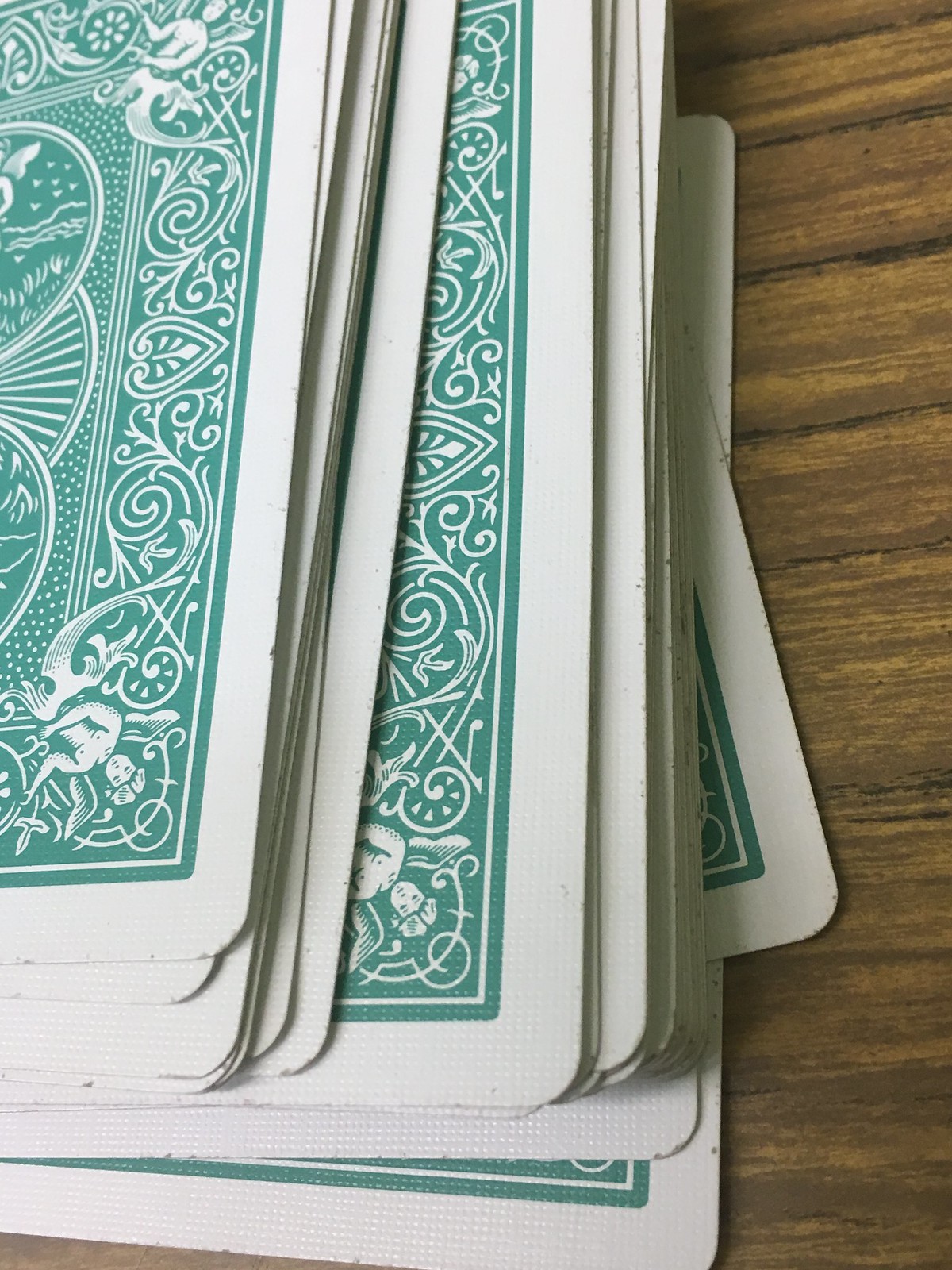An image depicting a pile of playing cards lies on a wooden table, whose surface is a rich brown adorned with subtle gold streaks running through the slats. The cards are disorganized, forming a casual heap in the bottom corner of the image. While the cards are not neatly aligned, their overall arrangement retains a somewhat piled structure.

The visible side of the cards displays a distinct design, featuring a textured white border that frames the interior of each card. The central portion of the card is a greenish-blue background embellished with various intricate white shapes. In the corner of each card, a small character illustration adds a whimsical touch to the overall visual theme. The focus remains solely on this decorated side of the cards, with none of the numbered faces or suits visible.